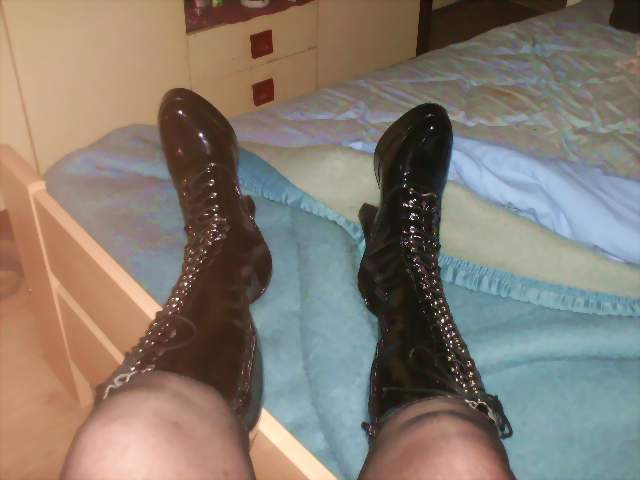This is a detailed photograph taken inside a bedroom, capturing a pair of fair-skinned legs wearing sheer black stockings and shiny black knee-high boots. The boots are adorned with silver-tone eyelets running all the way up from the foot to just below the knee. The feet are propped up on a bed, resting on a powder blue blanket with a satin edge. The mattress, partly exposed, features a whitish color and a mattress pad that is pulled back. The wooden bed frame is short and blonde, visible at the foot of the bed. In the background, there are white drawers with dark handles, a beige carpet, and some indistinct details possibly including a poster or a wall. The boots' glossy surface and the overall intimate setting add a stylish and cozy ambiance to the scene.